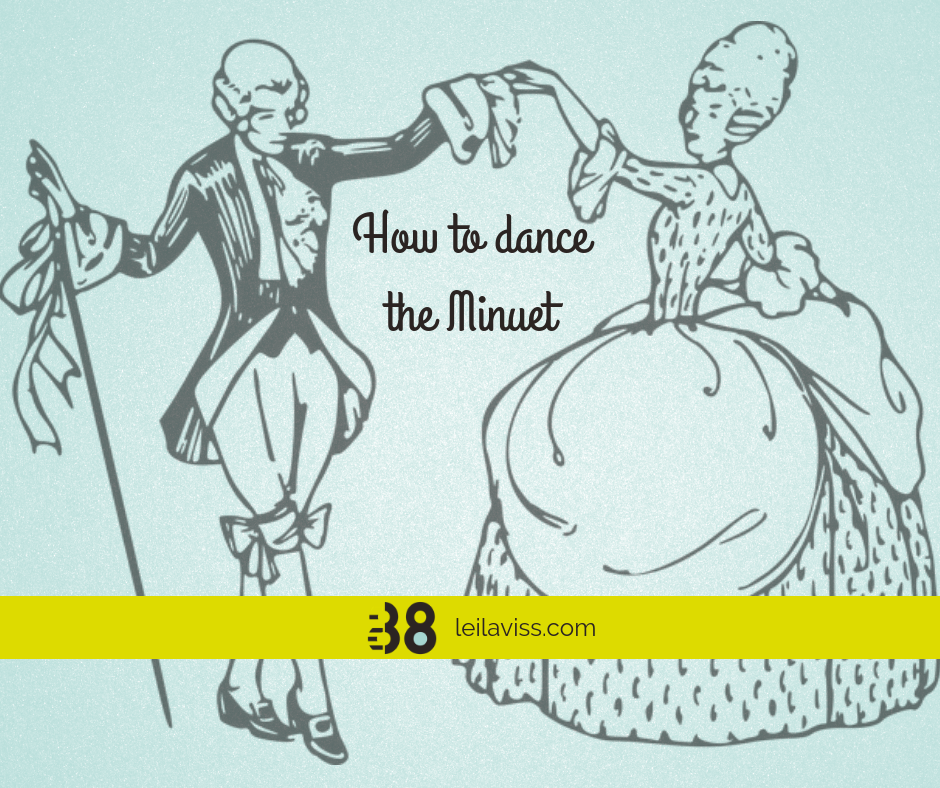The image features a detailed black drawing on a light blue paper backdrop, prominently displaying the text "How to Dance the Minuet" in elegant cursive at its center. To the left, it depicts a man adorned in colonial-era attire, including a long black jacket with extended cuffs revealing puffy shirt sleeves, knee-length bloomers with bows, long socks, and black shoes with buckles. His hair is styled in short tight curls on either side of his head, reminiscent of George Washington’s. He is holding a cane in his right hand and extending his left hand to a woman. The woman, dressed in a voluminous hoop skirt gown, has her hair intricately styled in a beehive wrap. They seem to be engaged in a dance, reflecting the minuet's elegant choreography. Below this central imagery, a thick yellow rectangle spans the bottom, inscribed with the number 88 and the website "LeilaVist.com," suggesting the image may serve as an informational or promotional graphic for learning this traditional dance.